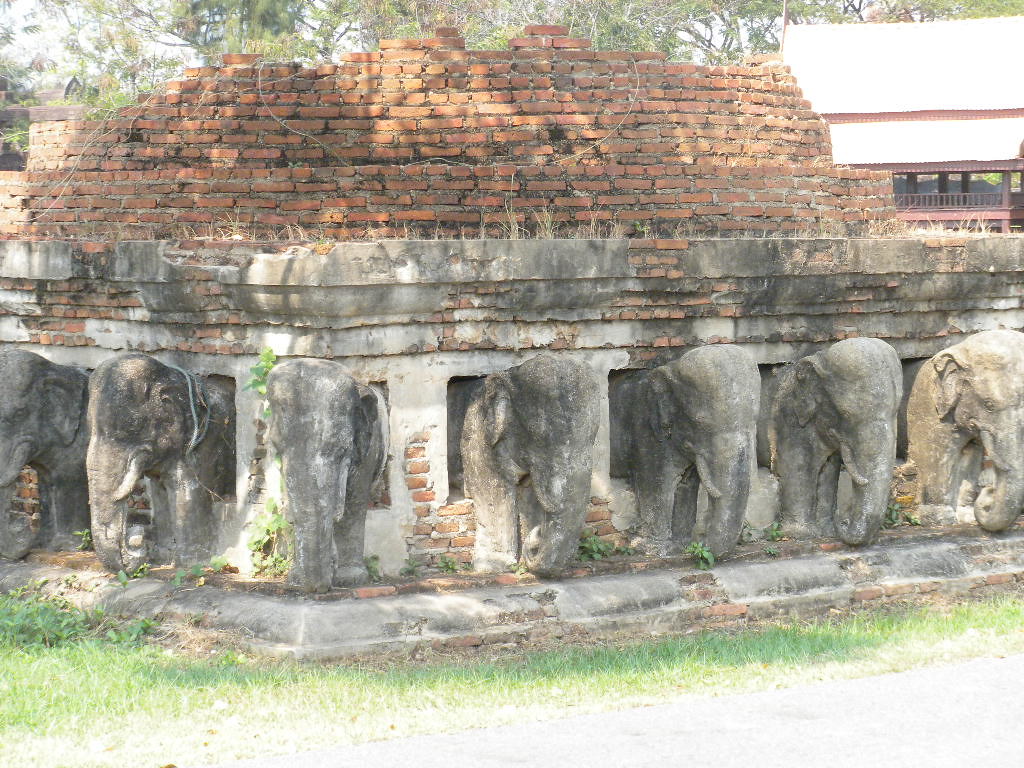The image depicts a very old, outdoor stone monument surrounded by lush green grass that becomes washed out due to sunlight reflections. The upper part of the photograph features a clear blue sky, thinly-leafed green trees, and a white, steep roof reflecting sunlight. The monument itself is made from concrete and bricks, with visible signs of age and wear including cracks and moss growth. Elephant heads, speckled with white and green from moss and dirt, are intricately carved around the base of the structure. There are six elephant statues facing outward towards the grass. The structure is rectangular, with an open area beneath the roof that lacks doors, allowing entry. The roof, composed of brittle-looking brown bricks, has small plants and weeds growing at its edges, emphasizing its ancient, weathered condition.